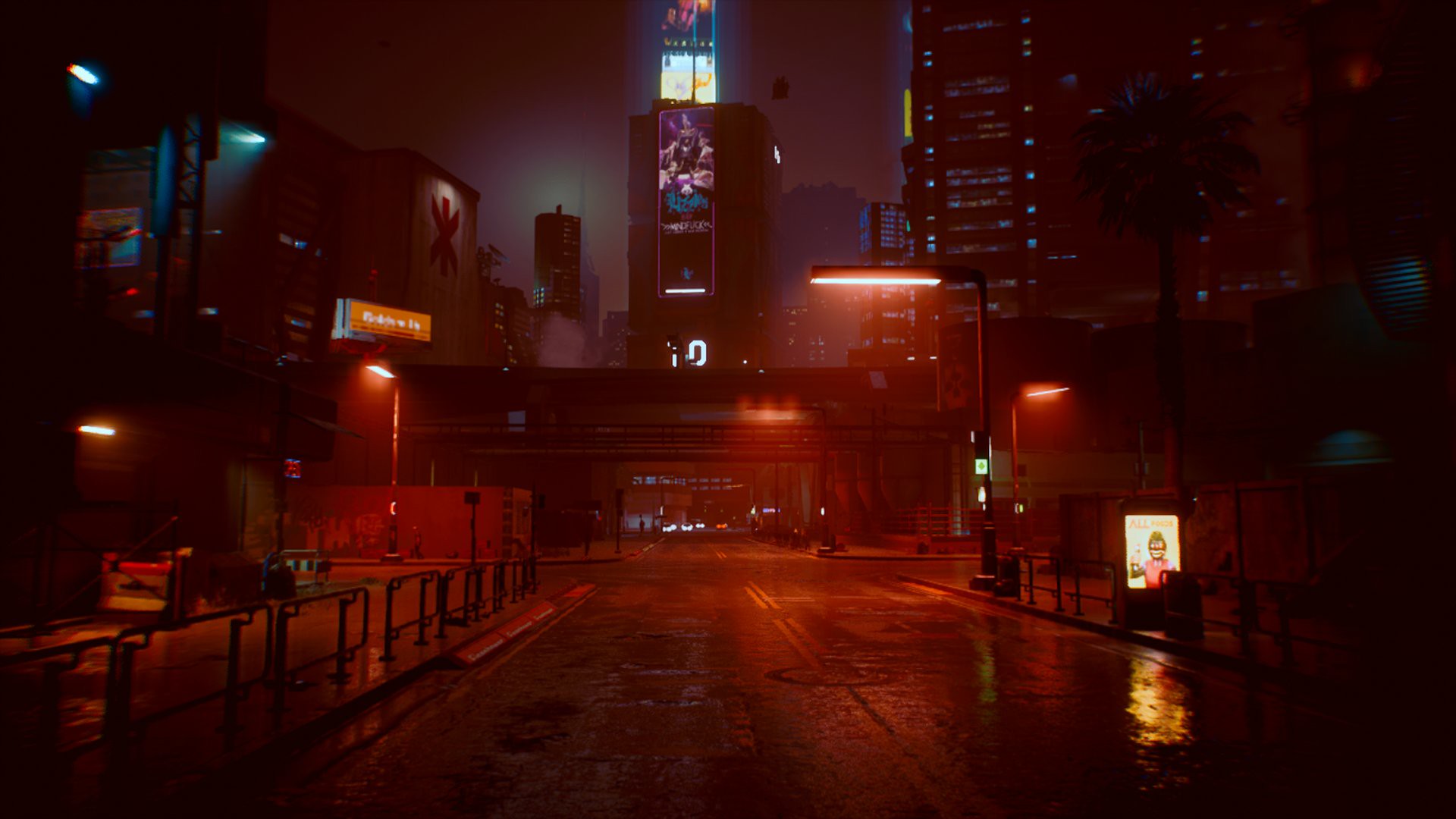This nighttime photograph captures a tranquil city street, devoid of immediate traffic but showcasing distant headlights. The street itself is illuminated by a series of glowing streetlights, casting a predominantly pink tinge across the scene, indicative of a wet surface reflecting the lights. Dominating the horizon is a city skyline filled with towering skyscrapers, each dotted with tiny, illuminated windows. Centrally prominent is a skyscraper featuring large, blue-glowing billboards, one of which displays an illuminated advertisement. To the left of the street, a metal fence lines the curb, near what appears to be a parked car. A bus stop and advertising signage are also noticeable under the soft glow of the streetlamps. Additionally, a tree silhouette and a reflective street sign enhance the depth and detail of the nighttime urban landscape. An overpass stretches across the street, adding another layer to this meticulously captured urban milieu. The overall scene is likely captured with a slow shutter speed, further intensifying the ambient light and pinkish hues enveloping the composition.